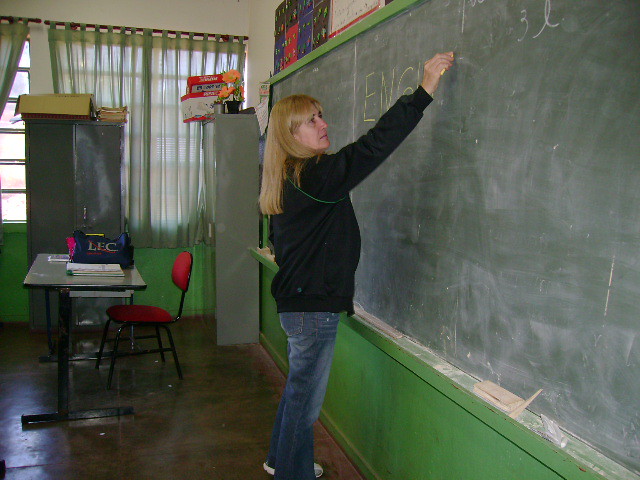The photo captures a detailed classroom scene centered around a teacher writing on a chalkboard with yellow chalk. The teacher, positioned prominently in the center of the image, is penning something that starts with the letters 'E' and 'G' on the board. She stands against a backdrop where the wall below the chalkboard is painted green, and the upper part is cream-colored. The floor of the classroom is wood, and to the left of the chalkboard, windows are adorned with green sheer curtains.

On the right side of the room, there's a teacher's table accompanied by a red padded chair, which has no arms. On top of the table sits a blue bag. Adjacent to the table are three filing cabinets, laden with papers and boxes. The color palette in the classroom includes shades of green, tan, brown, black, blue, red, orange, and gray, reflecting a typical indoor daytime setting.